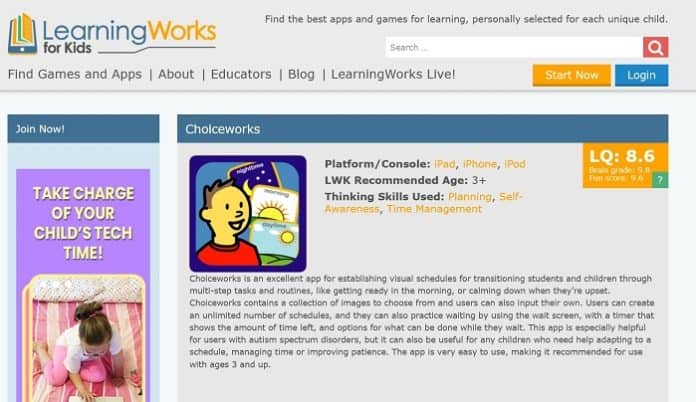The image features a light purple background. At the top, there is a yellow and green book icon set against a small blue background with a white dot beneath it. The text reads, "Learning Works for Kids," along with a slightly crooked line underneath. Below this, it states, "Find the Best Apps and Games for Learning Personally Selected for Each Unique Child."

Prominently, the image includes a search box with a small red box at the end, accompanied by additional text options like "Find Games and Apps," "About," "Educators Blog," "Learning Works Live," each with distinctive appearances. There is a yellow "Start Now" button and a blue "Login" button. At the top, there is a dark blue "Join Now" option.

The central content area also features a purple background with the text, "Take Charge of Your Child's Tech Time." An image of a small child playing on a pink and white striped blanket accompanies this text.

Another significant element is a large box titled, "Choice Works." This section features a small blue square showcasing a picture of a young boy, along with illustrations depicting a moon, stars, sunshine, and a field. This section provides detailed information such as:

- Platforms: Console, iPad, iPhone, iPod
- LWK recommended age: Three-plus
- Thinking skills used: Planning, self-awareness, and time management

In the upper right corner, there is a yellow box displaying "LQ 8.6," and in the bottom right corner, a green box with a question mark symbol is present. The description for "Choice Works" is included on a light blue background, delivering comprehensive details about the application.